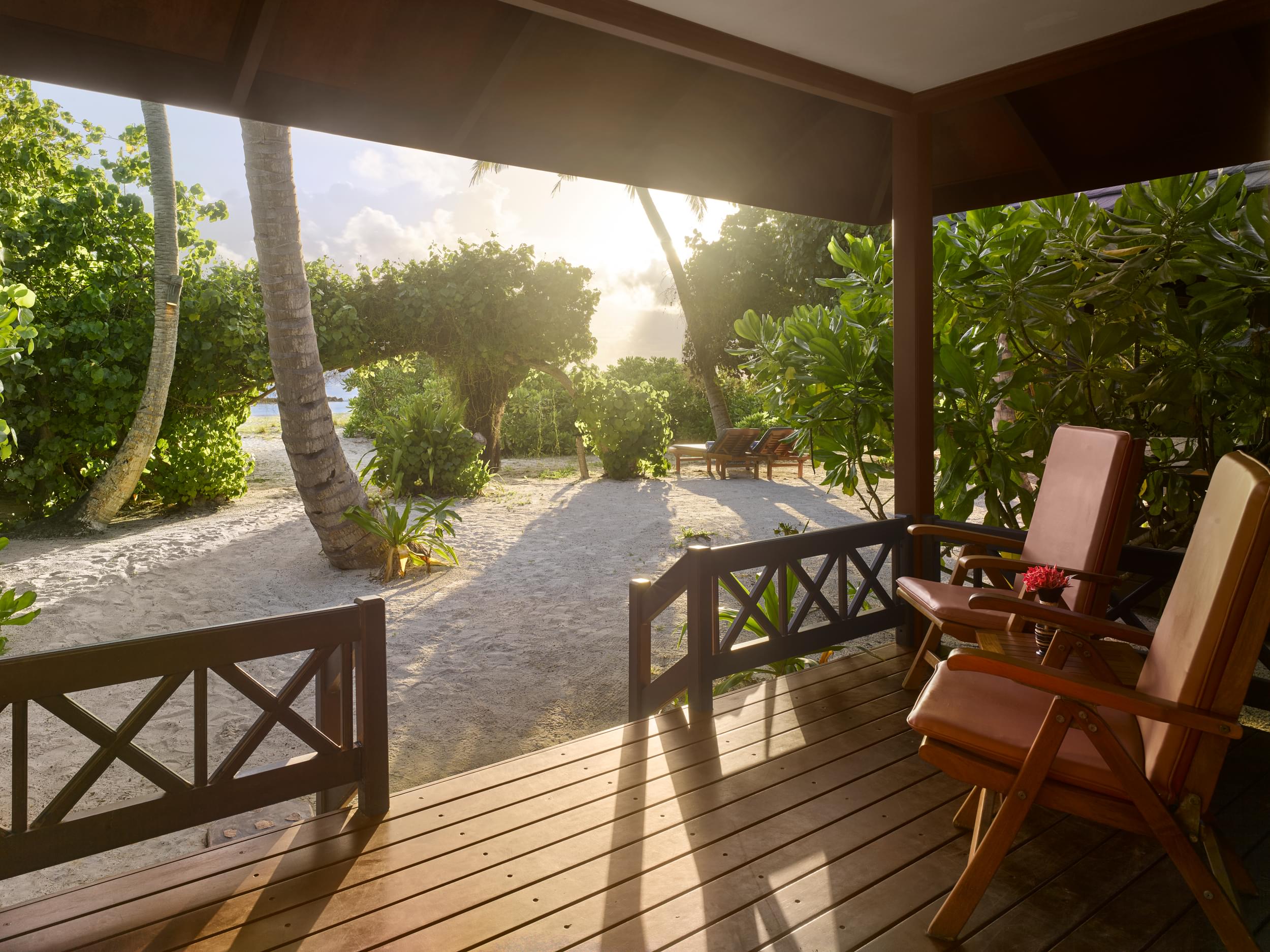The photograph captures a charming, covered wooden porch attached to a beachfront home. Situated in the lower right corner are two foldable wooden chairs, each adorned with orange cushions. Between the chairs rests a small wooden table holding a potted plant with vibrant pink flowers. The porch features a brown deck floor with a small raised wood barrier with X patterns and a gate leading down to the beach.

Beyond the porch, there is a sandy beach with several tall palm trees rising majestically. The scene is accentuated by lush greenery, including an elaborate bush structure that forms a natural archway, creating a picturesque transition from the yard to the sandy shore. The sky is visible overhead, with a few clouds illuminated by the sun. Additionally, lounge chairs can be seen scattered out on the sand, enhancing the tranquil atmosphere of this waterfront retreat.